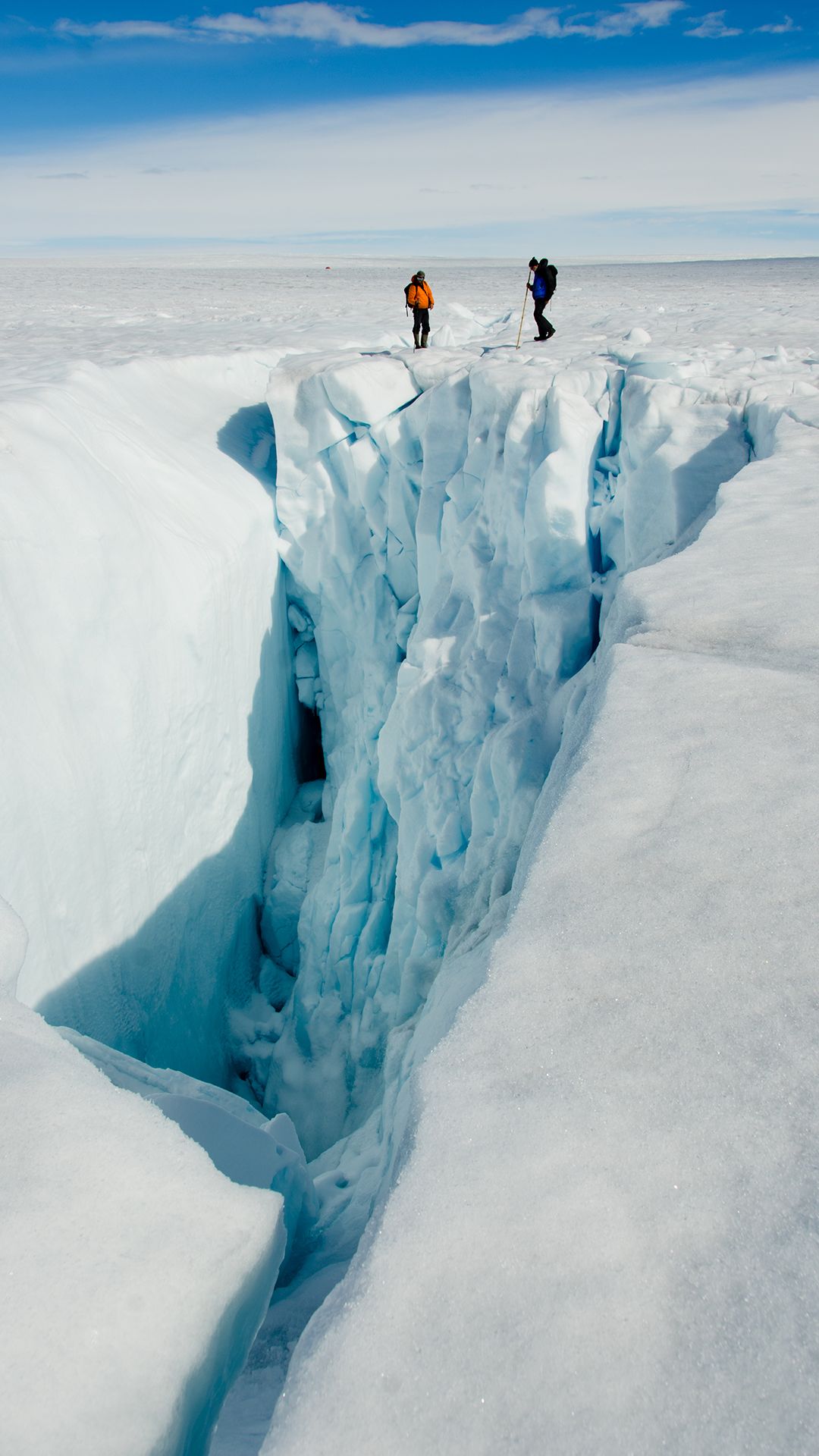The image is a color photograph capturing an awe-inspiring icy landscape, resembling the vast, barren expanses of the Arctic or Antarctica. Dominating the scene is a deep crevasse or ice canyon, possibly formed in a glacier, extending hundreds of feet into the ground, with its depths so profound they have taken on a blue hue from the accumulated snow and ice. Above this immense crevasse, a flat, solid ice plateau stretches towards the horizon. Two small figures stand at the edge of the crevasse, their size dwarfed by the sheer magnitude of the icy chasm. One explorer is distinct in a bright orange parka, while the other is equipped with trekking poles. The lack of facial details emphasizes the vastness of the environment that surrounds them. Above, a blue sky streaked with white clouds completes the upper quarter of the image, enhancing the desolate and untamed beauty of this frozen landscape.